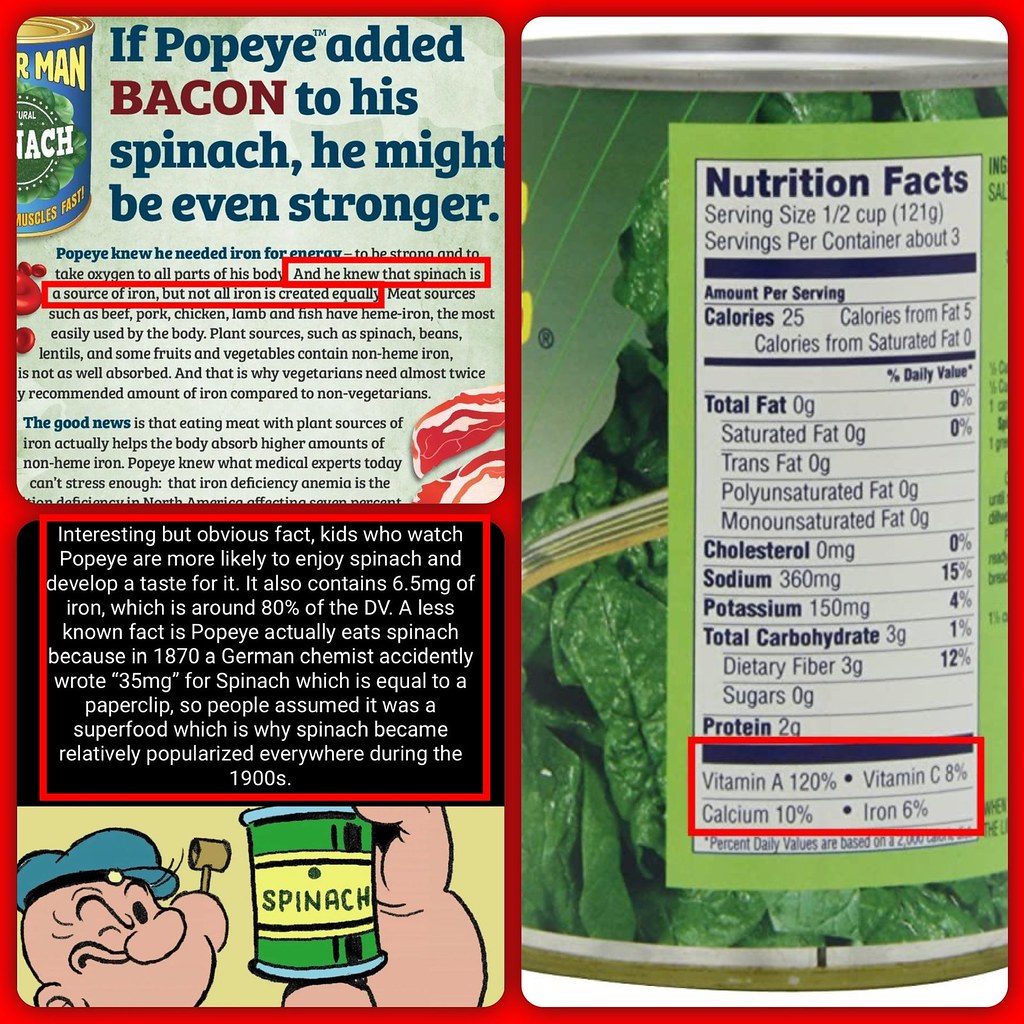The collage consists of three primary segments. On the right, a single image portrays a can of spinach, next to which a detailed "Nutrition Facts" label is superimposed in a green-framed white rectangle. Highlighted within the label is a red rectangle emphasizing the vitamin content: vitamin A at 120%, vitamin C at 8%, calcium at 10%, and iron at 6%. 

On the left, the collage features two images stacked vertically. The top image is an article suggesting that if Popeye added bacon to his spinach, he might become even stronger. Red rectangles within this article highlight key points, noting that Popeye knew spinach as a source of iron, yet emphasizing that not all iron is created equally.

Beneath this article, the bottom image shows a vintage cartoon depiction of Popeye holding a can of spinach. Positioned between the article and the Popeye image is another article, this one with white text on a black background. It discusses strategies for encouraging children to eat more spinach, specifically by letting them watch Popeye cartoons.

The overall layout effectively combines informative elements about spinach's nutritional benefits with engaging cultural references to Popeye, promoting healthier eating habits in an approachable manner.